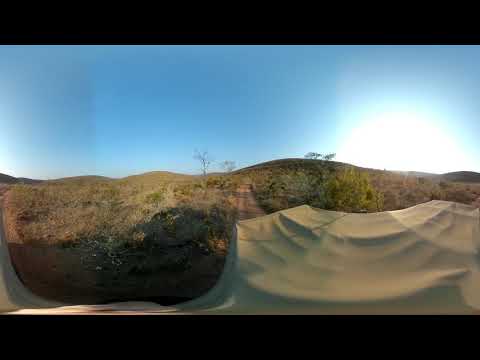This panoramic photograph captures a dry, expansive outdoor scene under a bright blue sky. The image is bordered on the top and bottom by black horizontal bands, creating a letterbox effect. Dominating the landscape are rolling hills covered in patches of green and brown grass, indicating varying levels of hydration. In the background, rugged mountains are faintly visible. A significant feature on the right side of the horizon is a white half-dome of light, suggesting the rising sun, which casts a bright glow across the scene. In the foreground, there is a tan tent that subtly dips on the left side and rises on the right, set against a sandy area. Scattered trees and bushes are also visible, although difficult to discern clearly due to the immense distance. Overall, the image evokes a sense of vastness and a slightly arid, grassy environment under a clear, bright sky.